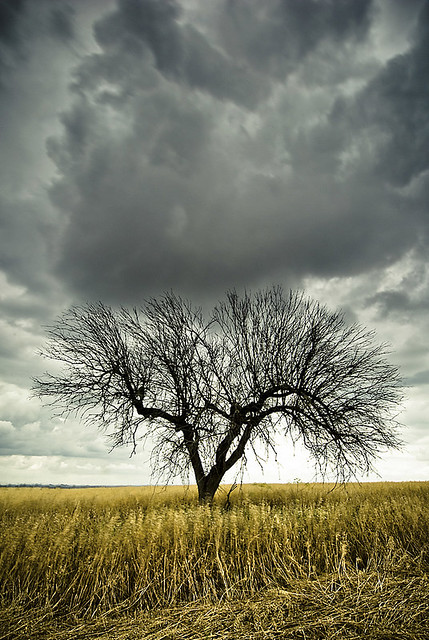A striking photograph captures the stark beauty of a barren tree standing alone in the midst of a vast, amber-colored wheat field. The tall grass, heavy with seeds at its tips, spans the foreground, though some of it appears flattened or distressed, suggesting a windblown or partially plowed landscape. The scene is enveloped by an overcast sky, dominated by dense, dark gray cumulonimbus clouds. Despite the foreboding atmosphere, there is a sliver of bright light on the horizon, where the sky subtly lightens to a near-white, offering a hint of contrast to the otherwise somber palette. The overall composition, with its muted yellows and grays, evokes a sense of desolate beauty and quiet melancholy.